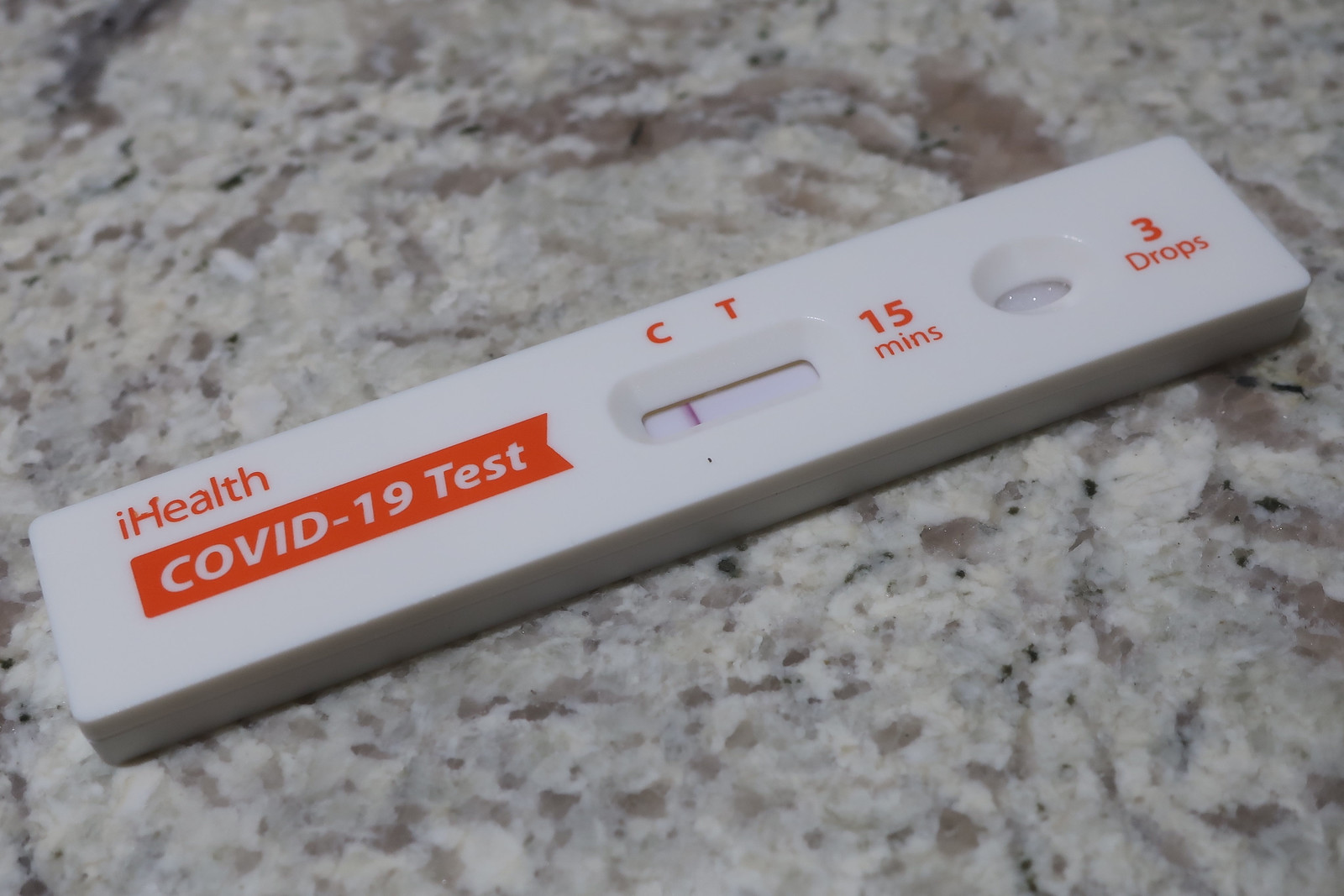A white granite countertop, adorned with subtle black specks and slight smears, serves as the backdrop for a diagonally placed COVID-19 test kit at its center. The kit, predominantly white with red text, features the words "Eye Health" positioned at the top left corner. Just below, the label "COVID-19 Test" is distinctly visible, accompanied by an indicative strip. Essential details include a black rectangular window in the middle, marked with letters 'C' and 'T' above it, alongside a vertical stripe descending through the window. 

To the right, an annotation reads "15 minutes," signaling the time required to check the results. The device also has an area designated for administering test drops, which appears to have already been used. The line below the 'C' confirms the test's validity by indicating that it is the control line, while the absence of a line beneath the 'T' designates a negative result, indicating that the individual does not have COVID-19.

The underside of the test is cast in shadow, suggesting illumination from the top that highlights the test kit. The text on the kit is mostly in red, enhancing visibility, except for the emphasized "COVID-19 Test" label. The overall lighting and positioning of the test kit ensure clear legibility of the results.